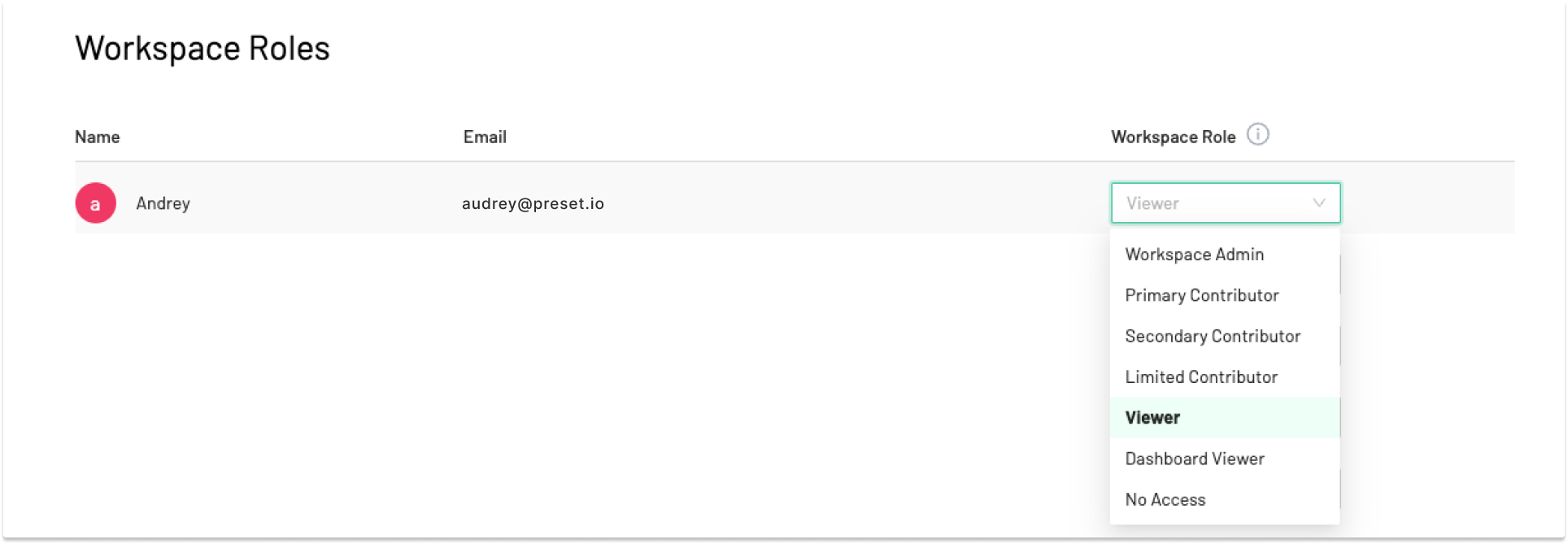The image depicts a page from a computer application, presented within a long horizontal rectangular window with a white background. In the upper left corner, bold black letters prominently display the words "Workspace Rules". Directly below this, a header section provides details about an individual, including their name, email, and workspace role. The header features a pink circle with a letter 'A' printed on it, which is associated with the name "Andre" written in black text beside the circle. Below the name, the email address "audrey@present.io" is listed. To the right of this email, a drop-down box is positioned under the workspace role category. The drop-down box, encased in a blue frame, contains the word "Viewer".